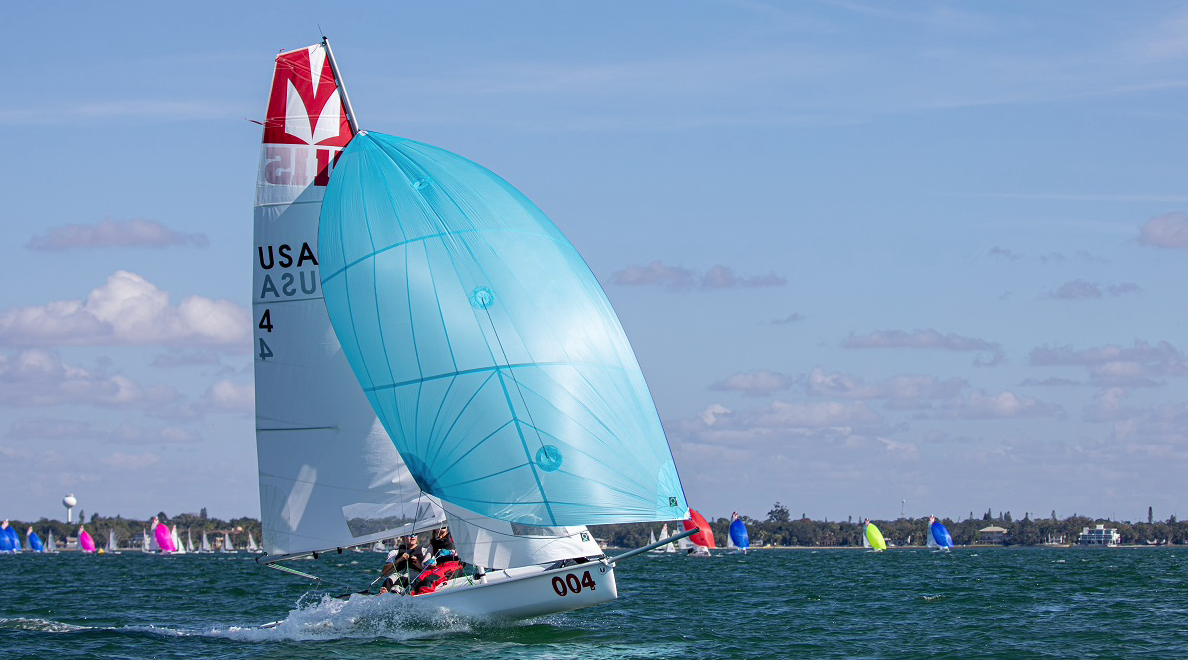In this image, you see a small sailboat navigating choppy, greenish-blue waters under mild weather with grayish-blue skies. The sailboat, positioned in the center of the photo, features two sails: a bright light blue front sail that is slightly domed due to the wind, and a larger white sail behind it with a red top featuring white leaf designs and "USA ASU 44" prominently displayed. Two people are aboard the vessel, leaning back and holding onto the sails as the front of the boat lifts slightly out of the water. In the background, the shoreline is lined with trees and numerous colorful sails in shades of blue, neon green, red, hot pink, and white, suggesting a lively boating competition.